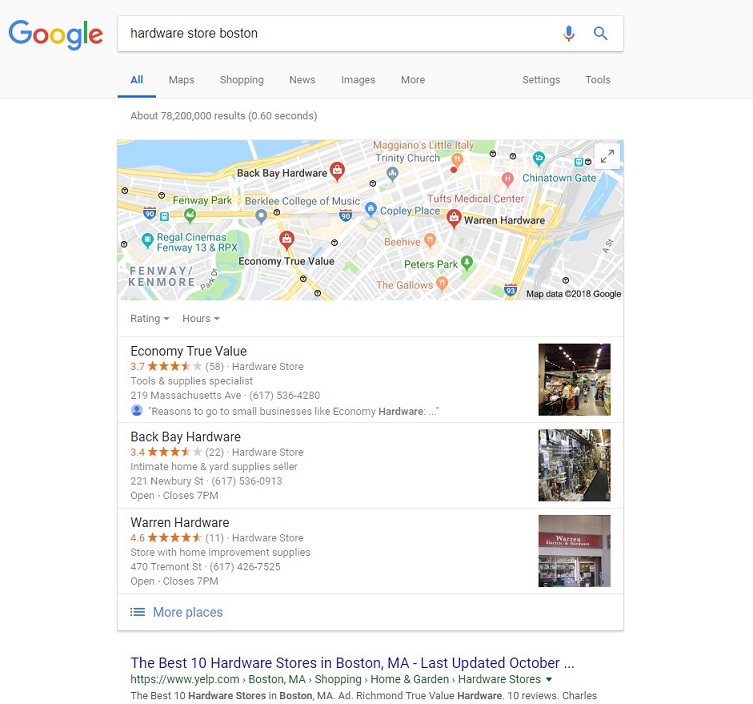This image is a screenshot of a Google search results page for "Hardware store Boston." At the top, there is the familiar Google search bar featuring the search term in black text. The search has returned approximately 78 million results.

Just below the search bar, a Google Maps snippet of Boston is displayed. The map shows the city's layout with yellow highways, gray buildings, and white roads. Several hardware stores are highlighted on the map. The first option listed is "Economy True Value," followed by "Black Bay Hardware" and "Warren Hardware."

Each store listing includes a rating highlighted in orange text along with a thumbnail image of the store on the right. Beneath these store listings, there is a blue hyperlink that typically leads to the store's website or relevant information, with the URL displayed in green text and accompanying black text providing additional context.